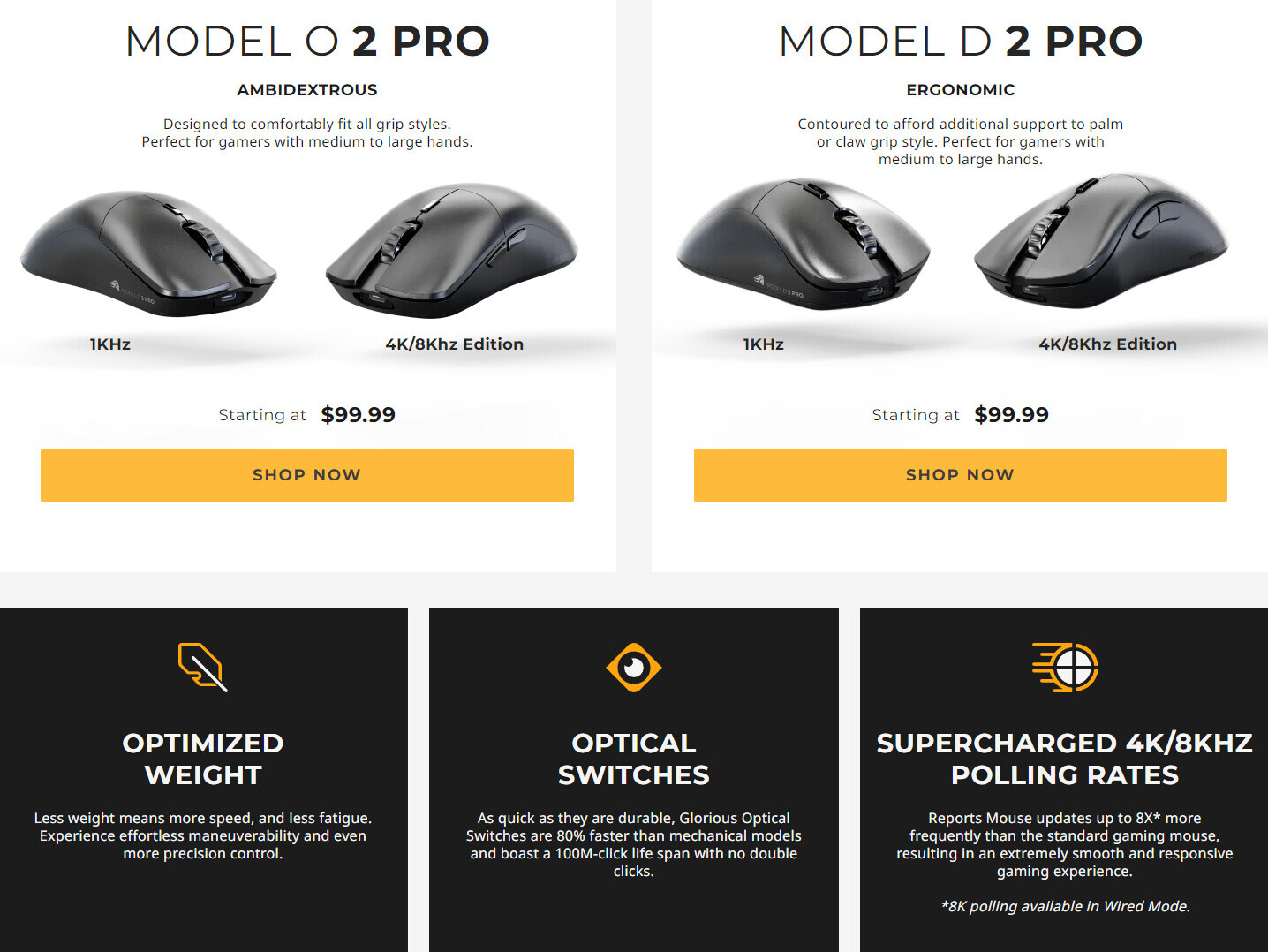The image is a screenshot of an Amazon webpage showcasing various models of computer mice. The background is a light gray, giving a clean and modern look. At the top, two distinct sections are displayed, each featuring different mouse models.

The left section highlights the "Model O2 Pro," prominently indicated in bold typeface. This ambidextrous mouse is designed to comfortably fit all grip styles, making it ideal for gamers with medium to large hands. The section features two mice: one facing right labeled "1k Hz," and another facing left labeled "4k/8k Hz Edition," starting at a price of $99.99. A golden "Shop Now" button is included for direct purchase.

The right section mirrors the layout but reviews the "Model D2 Pro." This mouse is ergonomically contoured to offer additional support for palm or claw grip styles, also suited for gamers with medium to large hands. The visual differences include a slightly wider design and a distinct mouse wheel. 

At the bottom, a couple of black boxes highlight key features shared by both models, including optimized weight, optical switches, and supercharged polling rates of 4k/8k Hz.